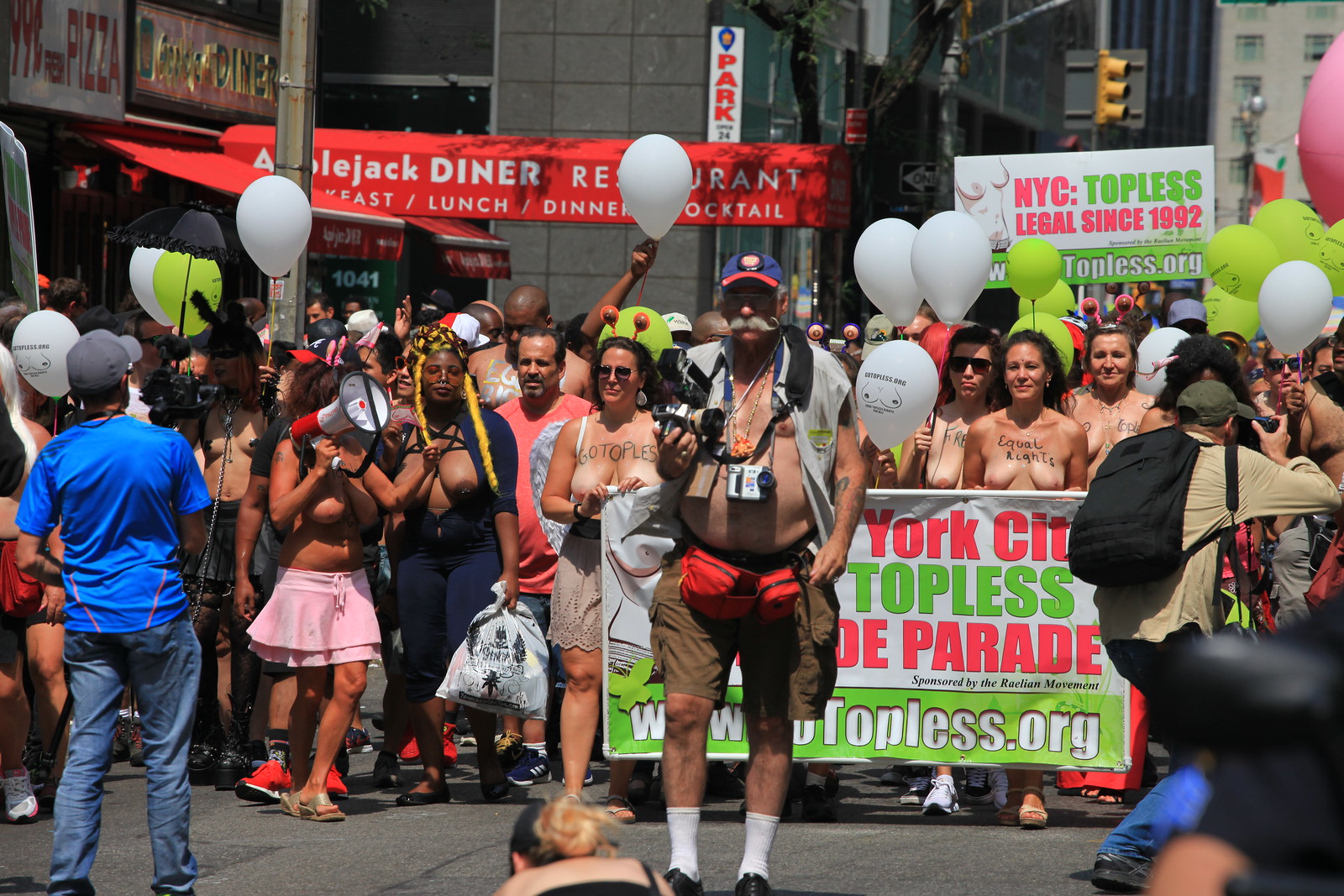In this vibrant, full-color outdoor photograph taken in broad daylight, a parade unfolds on a bustling street. Leading the procession is a man dressed in shorts, a top, and adorned with cameras and lanyards. Trailing behind him is a densely-packed group, predominantly women, who are topless. Though topless, none of the women appear fully naked. The crowd is diverse but predominantly white. Prominent signs and banners add context to the scene; one white sign features bright green and pink-red letters proclaiming, "NYC Topless Legal Since 1992," while another partially visible banner mentions "York Topless Parade" and "topless.org." The festive atmosphere is accentuated by an array of colorful balloons. In the background, city buildings loom, framing this unique parade promoting topless pride and the legality of public toplessness in New York City, apparently celebrating a legal history dating back to 1907. Photographers weave through the crowd, capturing the event from different angles.